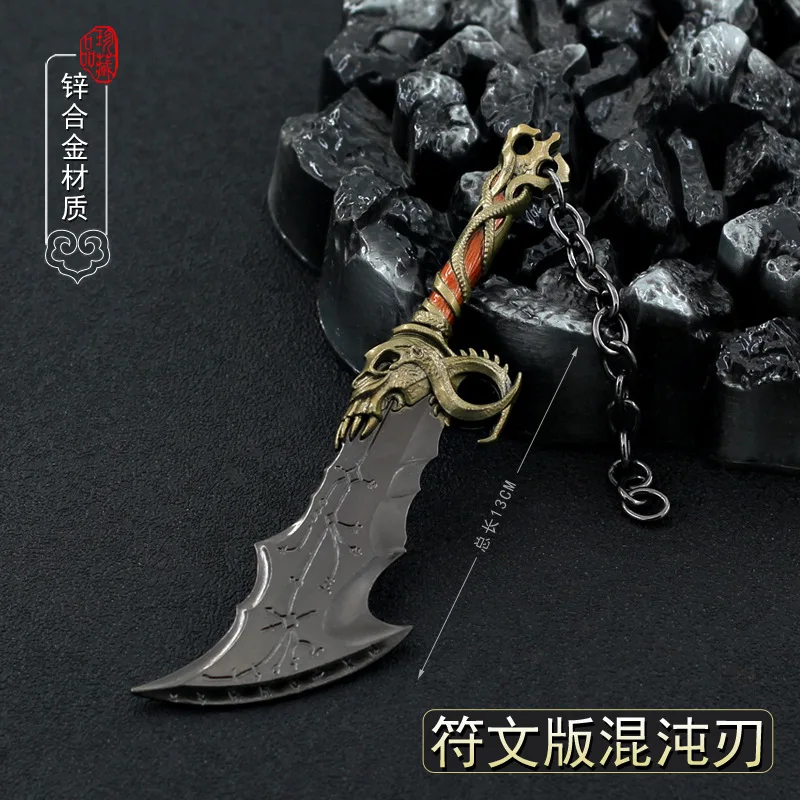The image showcases an intricately designed keychain in the form of a dagger or sword, artfully laid on a rugged black rock with various edges, all set against a solid black background. The dagger features a jagged and curved metallic black blade adorned with various hooks and spikes, culminating in a unique double-spiked tip. A red-orange plastic handle connects to the blade, and at the juncture, there are golden emblems of coiled serpents and a skull with sharp teeth, adding to the menacing aesthetic. The handle also features a silver chain. The photo includes Japanese text on banners in the top-left and bottom-right corners, with a red seal at the top of the upper banner. The text, along with the knife's measurements roughly described as “13 cm,” accentuates the detailed and exotic nature of the product.